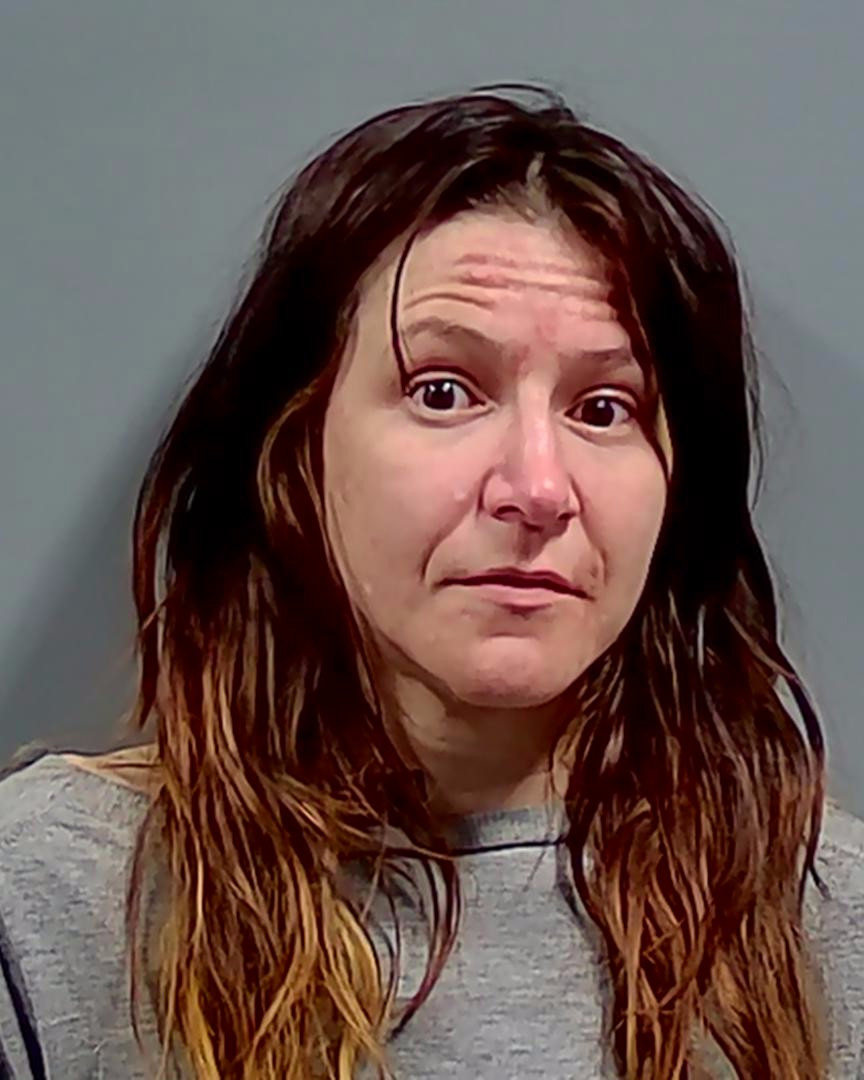This color photograph is a detailed close-up of a middle-aged Caucasian woman, focusing on her head and shoulders. She has light skin, with deep wrinkles marking her forehead and the area above her right eye (left side of the image for viewers). Her dark brown eyes appear arched and express a sense of unhappiness or possible trauma, though her mouth remains expressionless. Prominent wrinkles extend along the sides of her cheeks, which are themselves quite pronounced.

Her hair is long, slightly wavy, and parted in the middle, with a mix of dark brown and golden-blonde tones, creating a textured appearance. The hair looks either wet or possibly greasy. She is dressed in a grey top with a wide, high neckline. The backdrop is a plain grey with a subtle shadow cast on the left side, indicating a light source from the right.

The photo appears to be over-sharpened, perhaps for social media, which gives it a slightly unrealistic and hyper-detailed look. Overall, the woman's disheveled appearance and the detailed texture of the image suggest a moment captured under duress or deep thought.